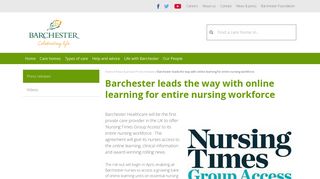Screenshot of a Barchester Web Page (Partial View)

The upper section of the page features a gray banner that spans the width of the screenshot. Just below this banner, in the upper left corner, there is an artistic leaf image or drawing. Adjacent to the leaf, the text reads, "Barchester, Celebrating Life." On the right-hand side, a rectangular, horizontally placed search box is prominently positioned.

Underneath the aforementioned elements is a thick green horizontal line with small yellow text at its left end, which is indecipherable due to its size. Below this, on the left-hand side, a shorter green rectangle contains similarly small yellow text that is unreadable.

To the right of this rectangle, green text reads, "Barchester leads the way with online learning for entire nursing workforce." Beneath this headline, centrally aligned gray text is visible but unreadable at this viewing scale. At the bottom of the screenshot, in bold black text, it reads, "Nursing Times."